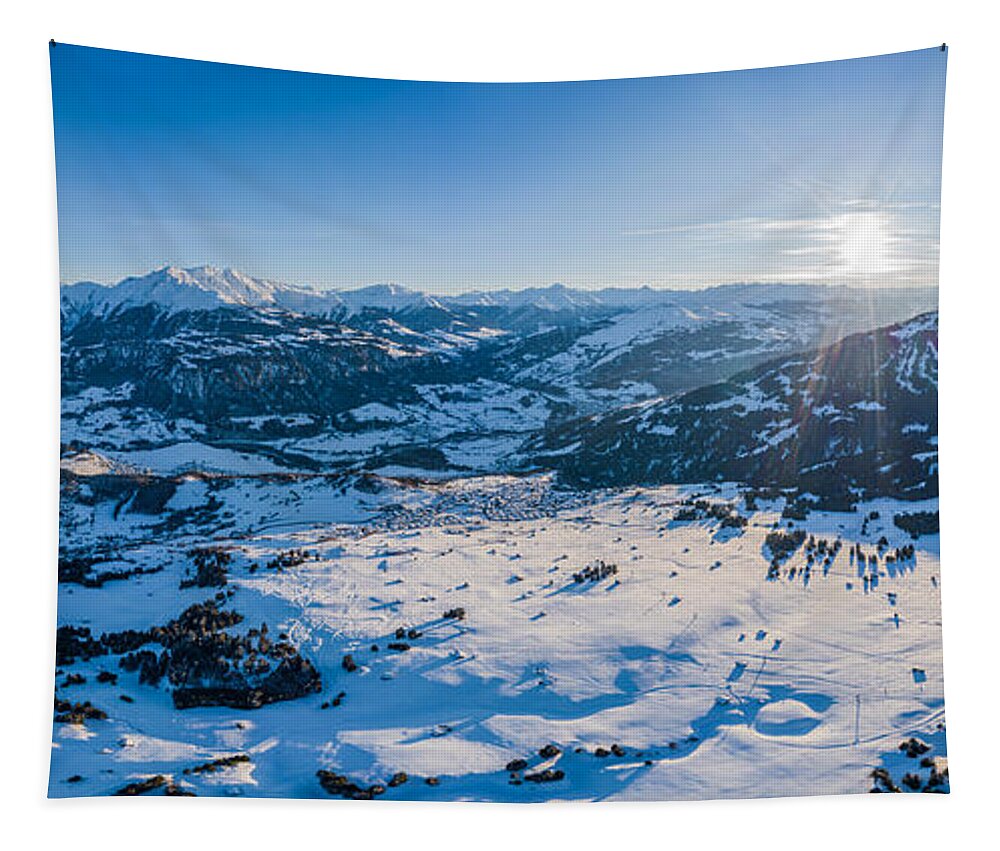A stunning winter aerial view captures a vast landscape of snow-capped mountains under a clear blue sky with the sun setting to the top right. The foreground features a relatively clear patch of snow, resembling a ski slope, dotted with scattered rocks and crisscrossed with well-defined ski lines. This area, devoid of trees, slopes gently up and down, interspersed with indents, hills, little gullies, and valleys. Dark rocky mountains dominate the foreground, their peaks completely covered in snow, while larger snowy mountains and smaller rolling hills stretch out into the distance. Dotted intermittently are small trees, adding texture to the snowy expanse. Hints of a distant village or buildings can be discerned far below. The sky transitions to a light gradient near the horizon, with sunbeams radiating upwards and downwards, casting a serene, almost ethereal glow over the winter landscape.